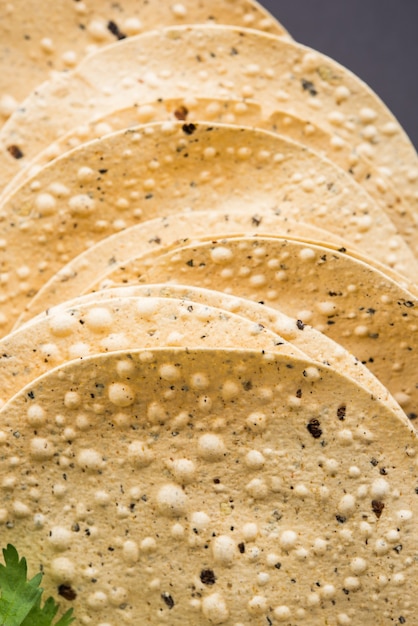The image is a close-up of approximately ten yellow-beige corn tortillas, arranged vertically in a feathered pattern from the top left to the bottom. Some of the tortillas are positioned higher than others, creating a staggered look. The tortillas are displayed with visible air pockets and dark spots, indicative of frying or baking. In the bottom left corner, there is a small piece of cilantro, adding a touch of greenery. The background is slightly blurry, emphasizing the detailed texture of the tortillas.